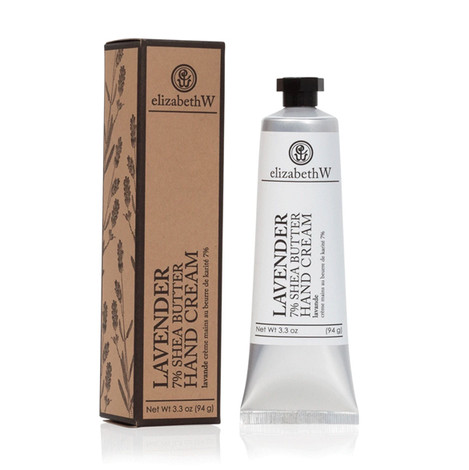This detailed photograph showcases a beauty product, specifically a hand cream, along with its packaging. On the left side of the image stands a vertically positioned light brown cardboard box with dark brown borders and botanical illustrations. The top of the box features the brand name and logo, "Elizabeth W," followed by the product name, "Lavender 7% Shea Butter Hand Cream," written vertically. The bottom portion of the box includes additional text indicating the product's net weight (3.3 oz/94 g). To the right of the box, the silver metallic tube of hand cream, capped with a black plastic top, is displayed. The tube bears a white label with the same branding and product details as the box. The clean, white background of the photograph emphasizes the packaging and product, allowing the details to stand out clearly.